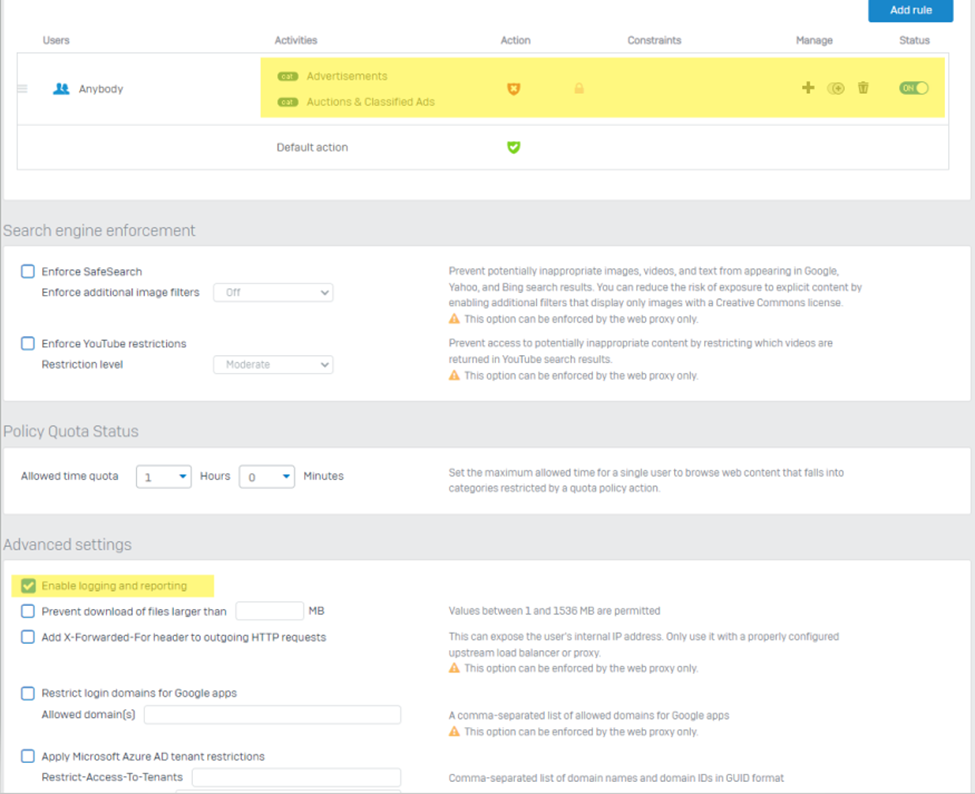Here is a cleaned-up and detailed caption for the described image:

---

The image depicts a comprehensive online form interface for managing user activities, advertisements, and other functionalities. At the top, the form headers include "Users", "Anybody", "Activities", "Advertisements", "Auctions and Classifieds", and "Action". There are two prominent shield icons: an orange shield with an X mark and a green shield with a check mark.

Under the "Constraints" section, options include "None" and "Manage". The interface features a circle with a plus sign for adding new constraints and a trash can icon for deleting them. The status field is highlighted in yellow and reads "On".

The next section is titled "Default Actions", indicating that default actions are active with a green check mark.

Further down, under the header "Search Engine Enforcement", there are various toggle options:
- Enforce Safe Search
- Enforce Additional Image Filters (with a dropdown menu, currently off)
- Enforce YouTube Restrictions (with a "Restriction Level" box which is not checked and has a dropdown set to "Moderate")

On the right-hand side, a detailed note explains the functionality: "Prevent potential inappropriate image, video, and text content from appearing in Google, Yahoo, and Bing search results. Reduce the risk of exposure to explicit content by enabling additional filters that display only images with Creative Commons licenses." A warning highlighted by a triangle with an exclamation point states: "This option can be enforced by the two web priority proxies only."

---
This revised caption provides a precise and clear description of each element in the image, making it easy to understand the content and structure of the form.